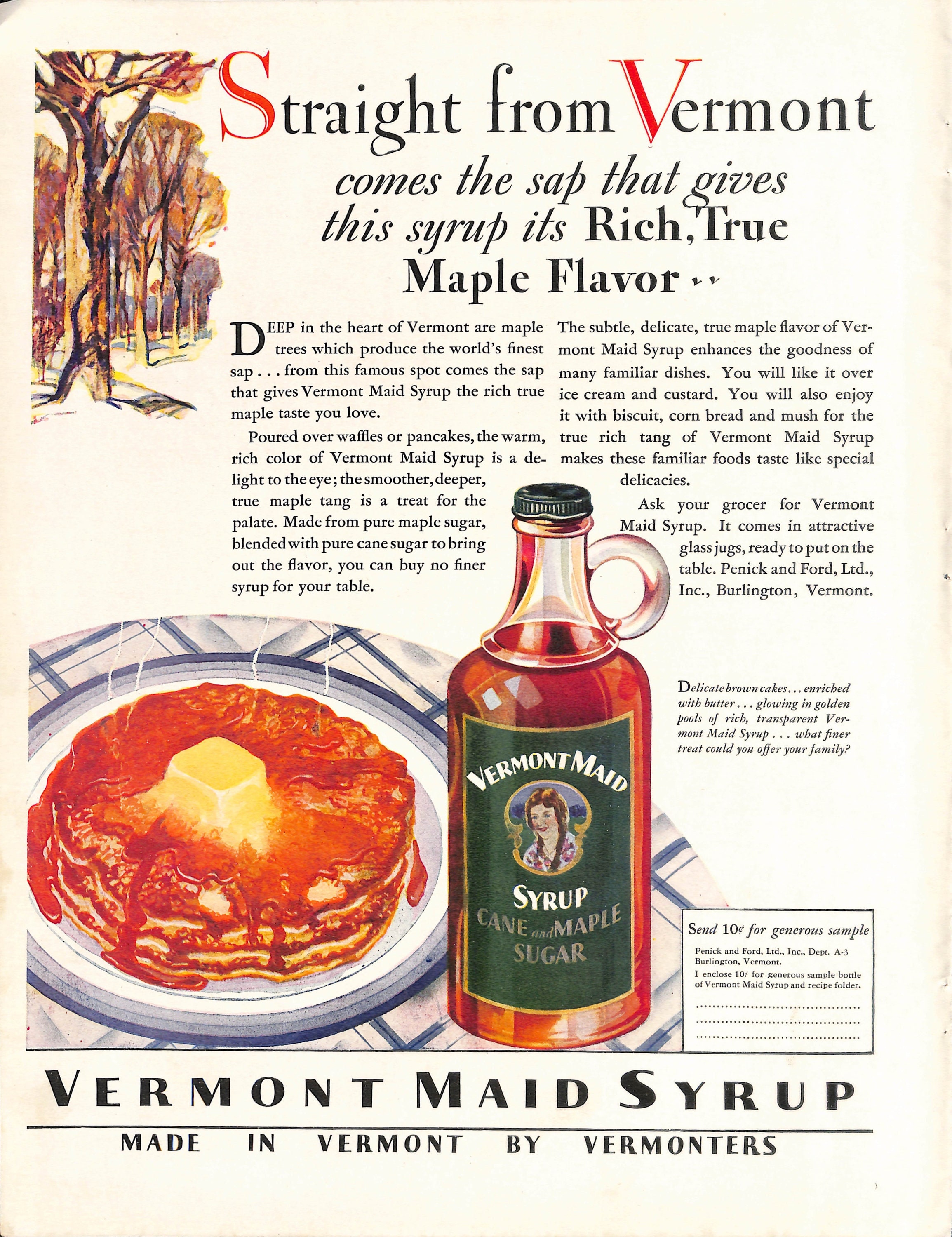This advertisement, likely a magazine cutout, showcases Vermont-made maple syrup with a central bottle prominently displayed. The bottle features a green label reading "Vermont Made," along with an image of a woman, and is inscribed with the words "syrup, cane, maple, sugar" near its base. To the bottom left of the bottle, a blue and white plate holds golden brown pancakes, enriched with butter, and draped in the rich, transparent syrup. The ad is embellished with a scenic painting of trees in the top left corner, hinting at the natural source of the syrup. The colors in the image include warm hues of brown, tan, yellow, and cooler shades of blue, green, with some white and a hint of red. Text at the top reads, "Straight from Vermont comes the sap that gives the syrup its rich, true maple flavor," with capitalized letters "S" and "V" in red. A paragraph below the title elaborates on the syrup's quality and authenticity. The bottom of the advertisement includes an offer, "Send 10 cents for a generous sample of Vermont-made syrup, made in Vermont by Vermonters."